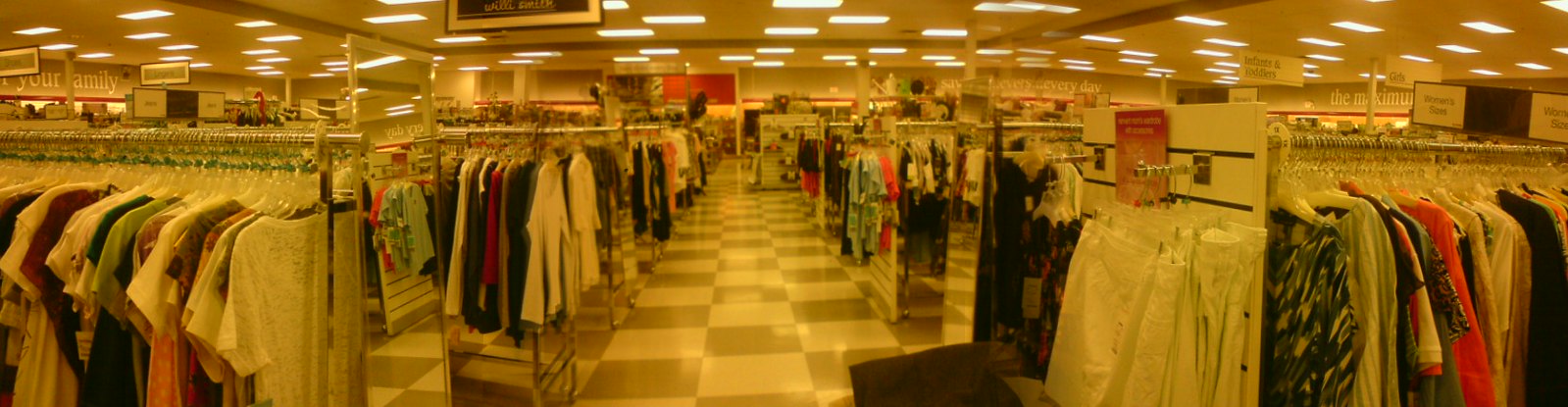This photograph captures the interior of a clothing store with a slightly distorted, stretched-out appearance, accentuated by an unusual yellow or golden hue, possibly due to aging or peculiar lighting. The store features a wide central aisle with a tiled floor in a shiny alternating pattern of large tan and ivory squares leading forward. Flanking this aisle are several racks of clothing, aligned horizontally to the viewer.

On the left side, approximately six racks are visible, predominately showcasing an assortment of tops like t-shirts, all neatly hung on clear plastic hangers. A mirror is positioned at the end of this row, contributing to the store’s functional setup. The right side hosts additional clothing racks, including a first rack laden with either pants or white skirts and some jackets. A small stool is placed in front of the first rack, suggesting a space for customers to sit or try on shoes. The store’s ceiling is a traditional drop ceiling fitted with fluorescent lights, further hinting at the photograph's vintage ambiance.